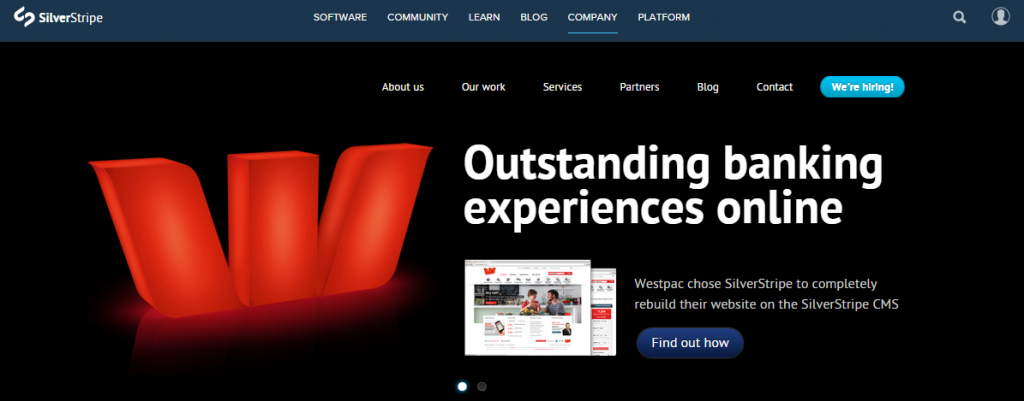"Silver Stripe's promotional image prominently features their tagline 'Outstanding Baking Experiences Online' alongside a bold red 'W' in the upper left-hand corner. The top section, nestled within a gray box, provides navigation options including Software, Community, Learn, Blog, Company, and Platform. Beneath this, a black box offers further clickable links: About Us, Our Work, Services, Partners, Blog, and Contact. A distinct blue circle with white text announces 'We're Hiring,' highlighting current job openings. The image also includes two visual representations of what appear to be webpages or calendar-like elements, emphasizing Silver Stripe's role in enhancing online banking experiences. The text encourages choosing Silver Stripe for a comprehensive website rebuild and invites users to 'find out how,' clearly positioning the company as a go-to platform for business solutions in online baking."